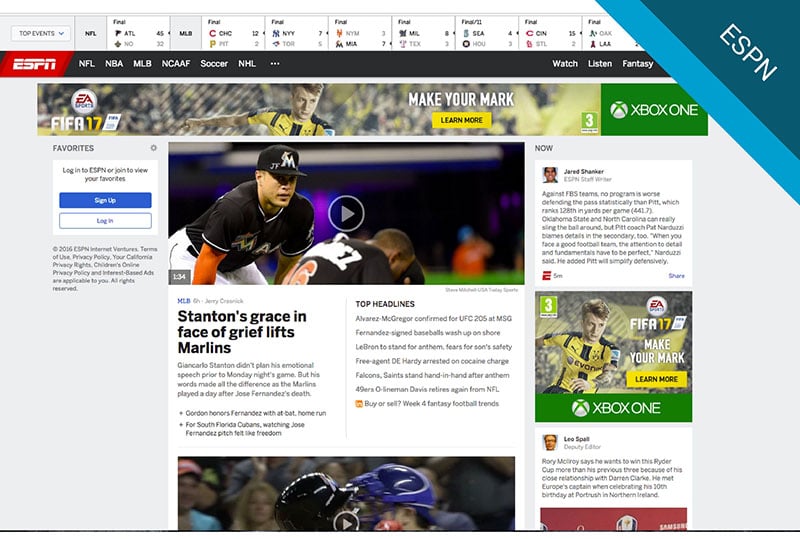This is a detailed screen capture of the ESPN desktop site's webpage.

**Upper Right Corner:**
- A small banner occupies the upper right corner. 
  - The upper part of the banner is dark teal blue with "ESPN" written in white lettering.
  - Below, the banner transitions to a light blue, highlighted by the title "Top Events" at the top, featuring various football and baseball scores.

**Main Navigation Bar:**
- Positioned slightly to the left, there's a prominent red banner with "ESPN" in white lettering.
  - Adjacent to this banner are menu options for NFL, NBA, MLB, NCAA football, soccer, NHL, and a hamburger menu.
  - To the right, the categories "Watch", "Listen", and "Fantasy" are displayed.

**Advertisements and Highlights:**
- Below the main navigation, there is an advertisement for FIFA 17 on Xbox One with the slogan "Make Your Mark." The ad features an image of a soccer player poised to kick a ball.

**User Interaction Section:**
- On the left, a section labeled "Favorites" includes an icon for settings.
  - Below this, there are prompts to "Login to ESPN or Join to view your favorites."
  - A blue bar with white text encourages users to "Sign Up," followed by a white bar with blue text for "Login."

**Headline and Image:**
- To the right, there's a picture of Giancarlo Stanton alongside another player, accompanied by the headline "Stanton's Grace in Face of Grief Lifts Marlins." This likely refers to the emotional period following Jose Fernandez's death.
  - Beneath this, an image shows a batter and catcher hugging, likely depicting Dee Gordon after hitting his home run in tribute to Jose Fernandez.

**Additional Content:**
- To the right, a small section labeled "Now" presents another article.
- Below all of this, there are further advertisements, including another one for Xbox One, and additional content relevant to golf.